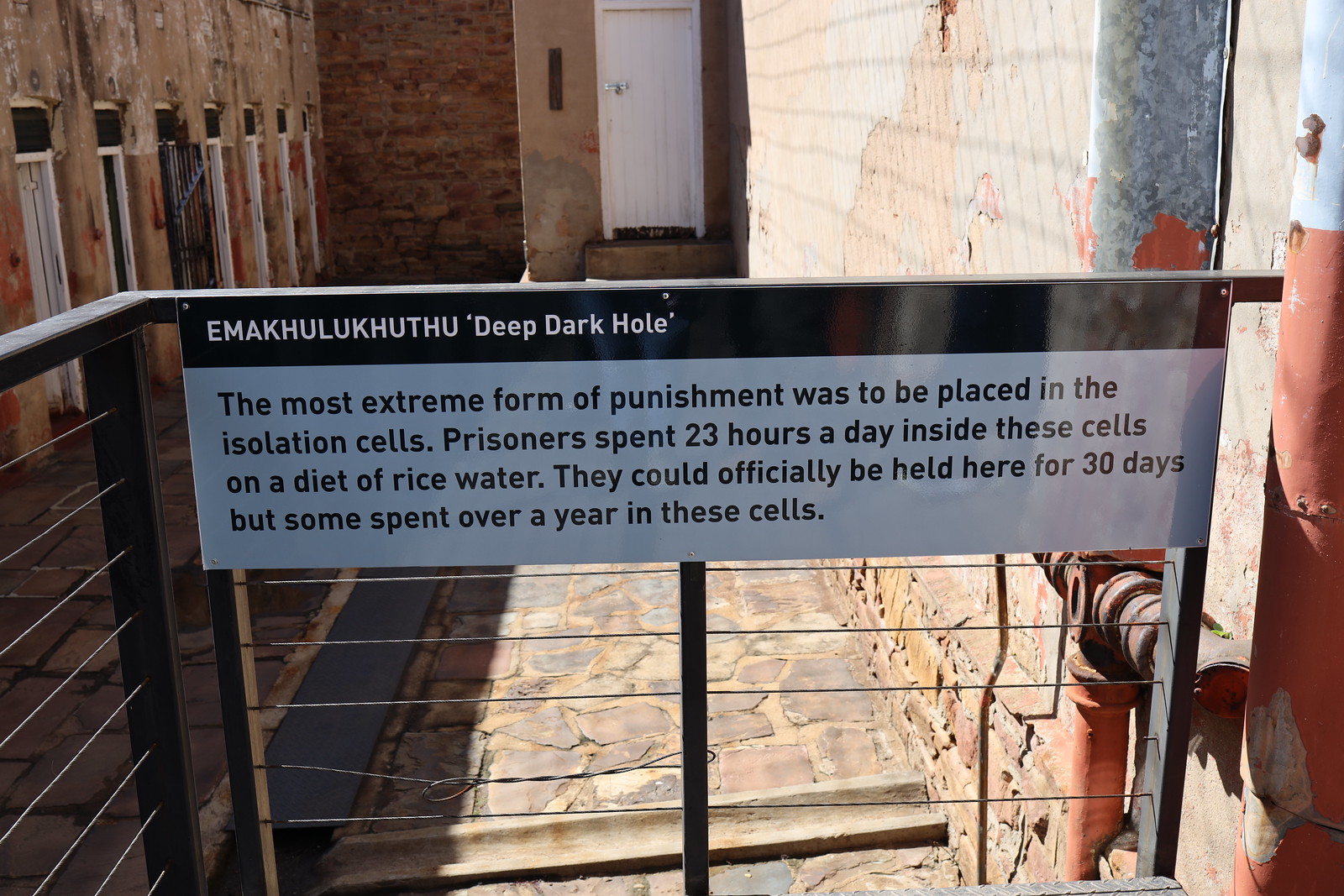This detailed color photograph centers on an informational plaque affixed to a metal gate, which is part of a larger metal fence with a gate. Beyond the gate, there is a stone wall, a stone floor, and windows with metal bars. The sign reads, "EMAKHULUKHUTHU - Deep Dark Hole. The most extreme form of punishment was to be placed in the isolation cells. Prisoners spent 23 hours a day inside these cells on a diet of rice water. They could officially be held here for 30 days, but some spent over a year in these cells." The scene depicts an area of a prison noted for its severe isolation cells. Additional details include visible pipes on the walls to the right and a color palette of brown, white, black, and silver. The photograph was taken during the daytime, and we are looking directly at the sign.